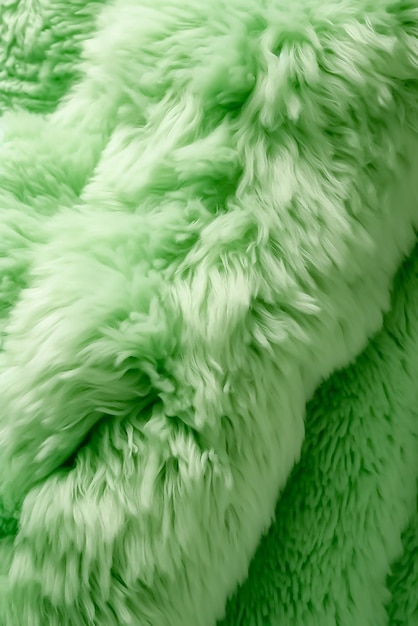The image is a detailed close-up photo of a bright, mint green, and very fuzzy stuffed animal or possibly a blanket with thick, fluffy fibers. The material appears well-loved with some matted sections, suggesting it has been frequently handled or carried around. The lighting in the photo highlights the thickness and fluffiness of the fur, giving it a fresh and vibrant appearance. The color is a refreshing shade of mint green, and the texture looks soft and inviting.